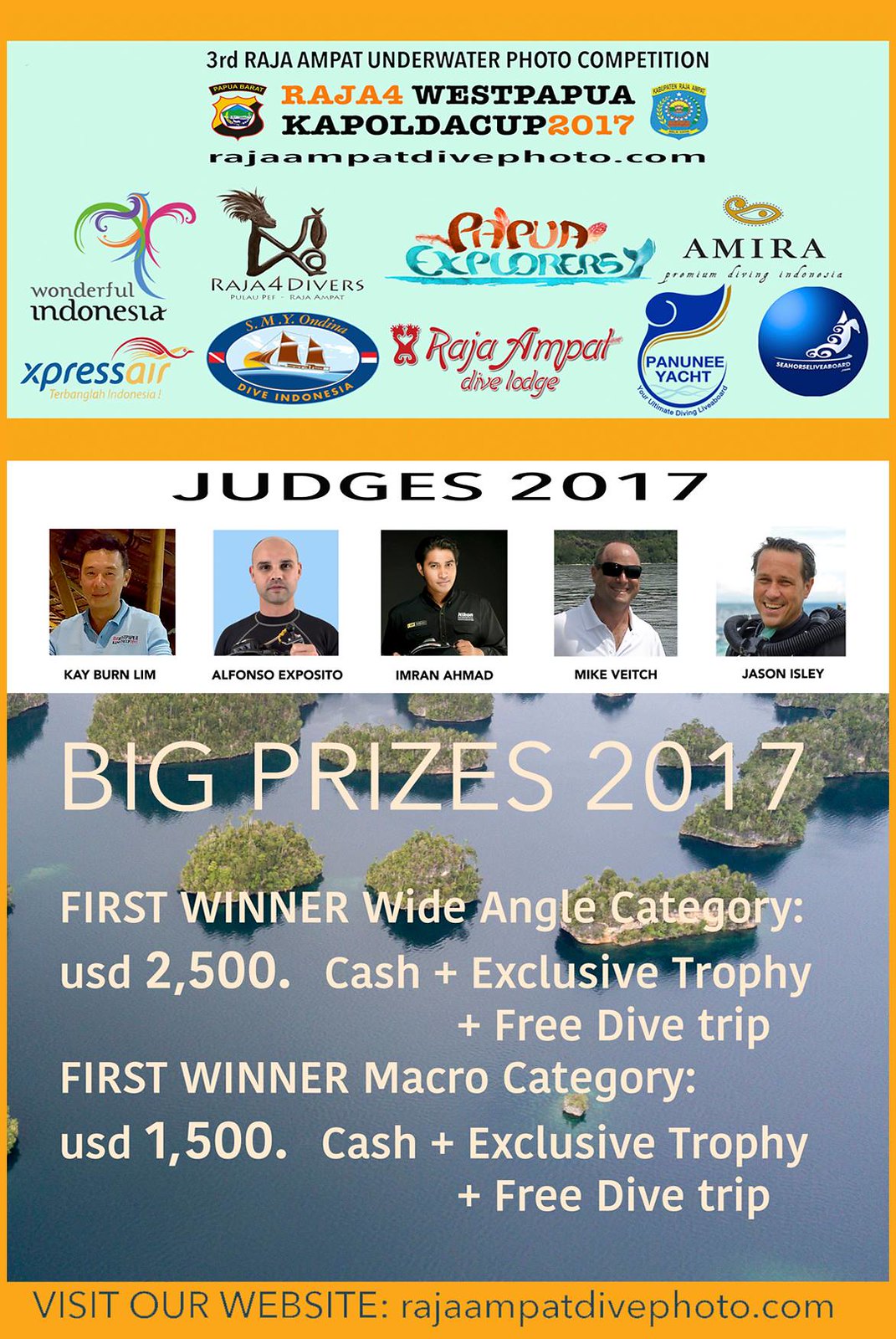This image is a tall, rectangular advertisement poster framed in an orange border. At the top of the poster is a wide, seafoam green rectangle, adorned with colorful logos from various businesses such as Wonderful Indonesia, Express Air Dive Indonesia, Raja for Divers, Amira Premium Luxury, Amira Premium Diving Indonesia, Panuni Yacht, Raja Ampat Dive Lodge, Pupua Explorers, and Simos Live Aboard, indicating sponsorship for the event. 

In black font at the top of the poster, it reads: "Third Raja Ampat Underwater Photo Competition, Raja IV West Papua Kapolda Cup 2017," followed by "rajampatdivephoto.com" in smaller text. Below this, a white rectangle features photographs of five men identified as the judges for 2017: Kayburn Lim, Alfonso Exposito, Imran Ahmad, Mike Veach, and Jason Isley. 

Further down, the poster showcases a scenic image of water with several small islands, overlaid with detailed text about the prizes. It reads: "Big Prizes 2017, First Winner Wide Angle Category: USD $2,500 Cash, Plus Exclusive Trophy, Plus Free Dive Trip; First Winner Macro Category: USD $1,500 Cash, Plus Exclusive Trophy, Plus Free Dive Trip." 

Finally, at the bottom of the poster, in all capital, dark gray font, it instructs viewers to "Visit our website: rajampatdivephoto.com."